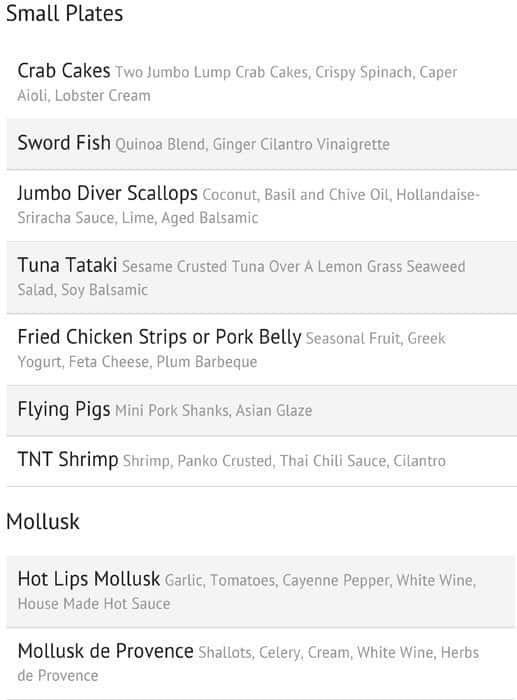**Menu: Small Plates**

1. **Crab Cakes**  
   Two jumbo lump crab cakes, served with crispy spinach, Keeper by Aioli, and lobster cream.

2. **Swordfish**  
   Accompanied by a quinoa blend and ginger cilantro vinaigrette.

3. **Jumbo Diver Scallops**  
   Highlighted with coconut basil and chive oil, hollandaise sriracha sauce, lime, and aged balsamic.

4. **Tuna Tataki**  
   Sesame-crusted tuna over a lemongrass seaweed salad, drizzled with soy balsamic.

5. **Fried Chicken Strips or Pork Belly**  
   Served with seasonal fruit, Greek yogurt, feta cheese, and plum barbecue sauce.

6. **Flying Pigs**  
   Mini pork shanks with an Asian glaze.

7. **TNT Shrimp**  
   Panko-crusted shrimp tossed in Thai chili sauce with cilantro.

---

**Mollusk**

1. **Hot Lips Mollusk**  
   Prepared with garlic, tomatoes, cayenne pepper, white wine, and house-made hot sauce.

2. **Mollusk de Province**  
   Featuring shallots, celery, cream, white wine, and herbs de Province.